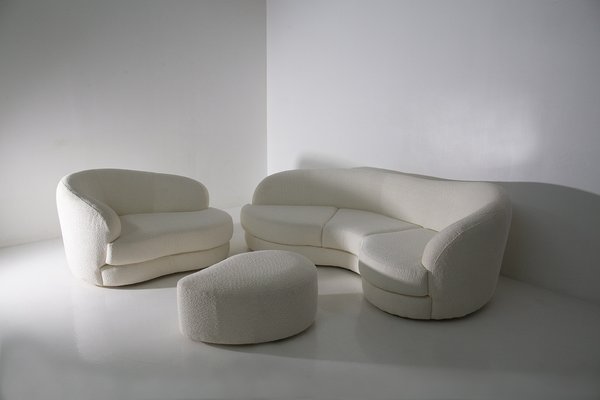This photograph features a minimalist room with a distinctively contemporary white furniture set. The room's walls, floor, and all the furniture are stark white, though the overall appearance shifts to various shades of gray due to the interplay of light and shadow, likely from a natural light source behind the camera. The setup includes a long, curvy, bean-shaped sofa with three seat cushions situated against the right wall. Its back is gently sloped and curves downward at the arms, blending modern aesthetics with soft contours. On the left side of the room is a smaller loveseat, featuring a single cushion and one armrest on the left side, suggestive of a chaise design. Centrally positioned is a teardrop or oval egg-shaped ottoman, matching in height and fabric style with both seating units. The floor is solid white and glossy, while the walls are matte and bare, creating a stark, open atmosphere. Bright light casts distinct shadows of the furniture, emphasizing the room's clean lines and serene, uncluttered space.